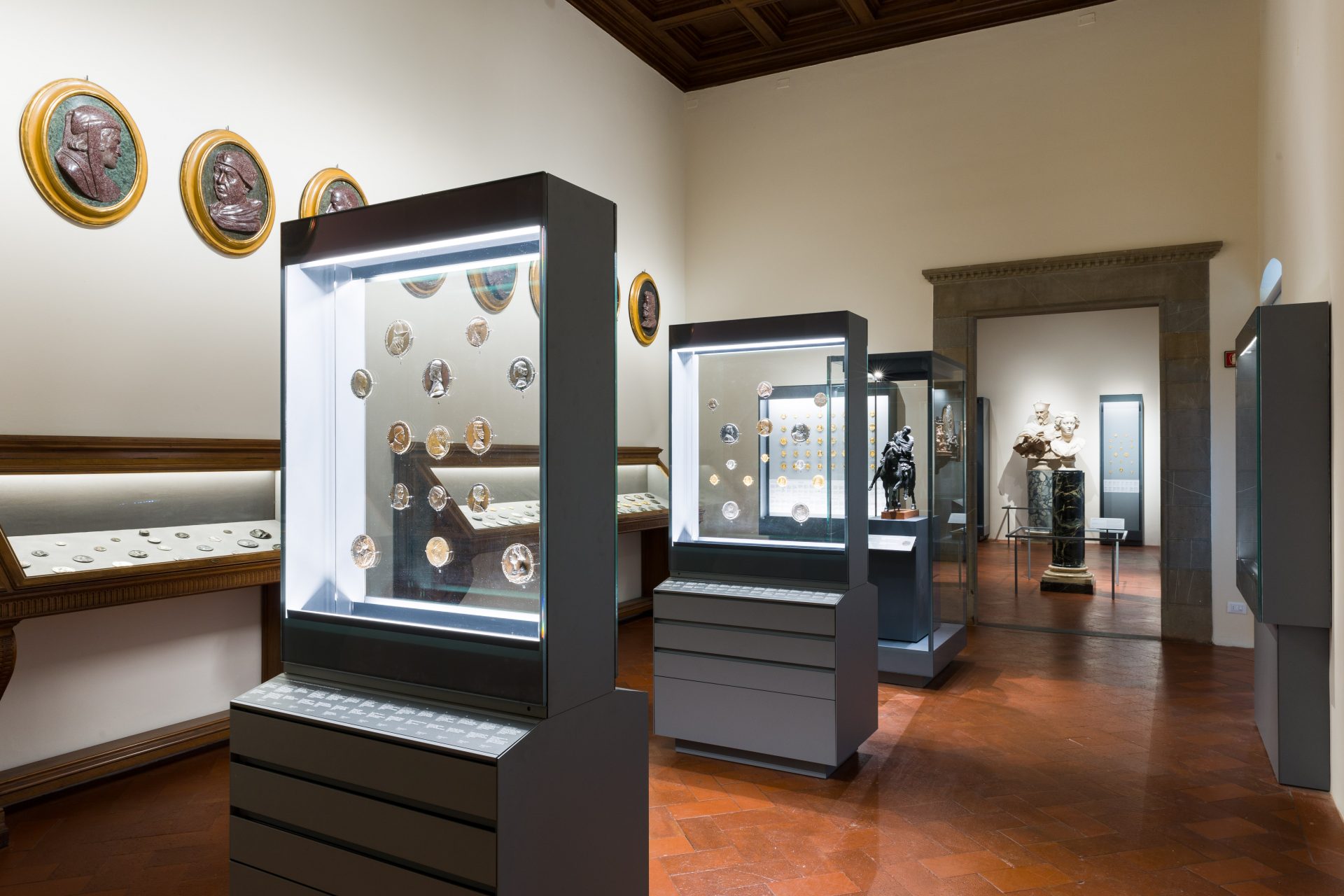This photograph captures the interior of a museum, exhibiting a well-curated array of historical artifacts. Dominating the center of the room are four tall display cases with thick glass enclosures, showcasing a collection of coins and military medals. Two of these cases are positioned in a row, flanked by a rectangular case featuring a statue of a man on a horse. The display cases are framed in black and surrounded by cherry wood, adding a touch of elegance to the high-ceilinged space. The shiny brown wooden floor reflects the ambient lighting, enhancing the grandeur of the exhibits.

On the walls to the left and right, large circular artworks—possibly reproductions of medals featuring bronze faces—are meticulously arranged, emphasizing the historical significance of the items. These wall displays extend from the top to the bottom, creating a continuous visual narrative. The walls are painted white, offering a stark contrast that highlights the exhibits.

At the far end of the room, a rectangular archway with gray trim opens into an adjoining space where statues on pedestals, including busts of a man and a woman, are visible, hinting at further exhibitions beyond. This connected room continues the museum's theme of showcasing significant historical artifacts, providing visitors with a comprehensive and immersive educational experience.